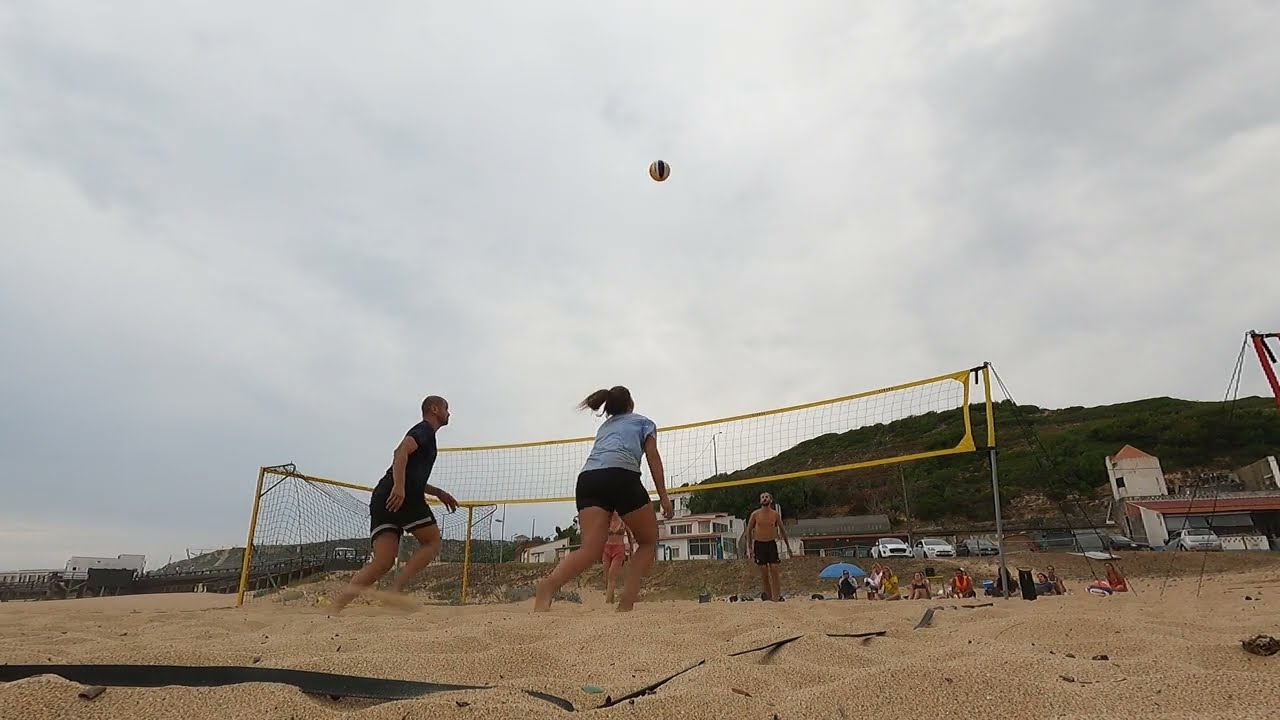The image depicts an intense beach volleyball game from a ground-level perspective, slightly angled upwards, with a lineup of players across the frame. In the foreground, closest to the camera and positioned in the bottom right corner, stand two players: a man on the left wearing a black t-shirt and black shorts and a woman on the right in a white or bluish t-shirt with black shorts, her hair tied in a ponytail. Both players are in a ready position, knees bent and eyes fixed on the ball above them, prepared to receive it.

The volleyball net, a prominent yellow streak across the middle of the image, separates the teams. On the opposing side, a shirtless man in black shorts stands near a woman in a bikini top and pink shorts, both more upright as they anticipate the ball. The background features a series of buildings with a lush, grassy hillside and a mountain further in the distance, adding depth to the scene. The sky dominates two-thirds of the composition, filled with layers of gray clouds, signaling an overcast day. Additional elements like a dock or pier are visible to the left, with beachgoers and some tents scattered in the distance, further enhancing the lively beach atmosphere.